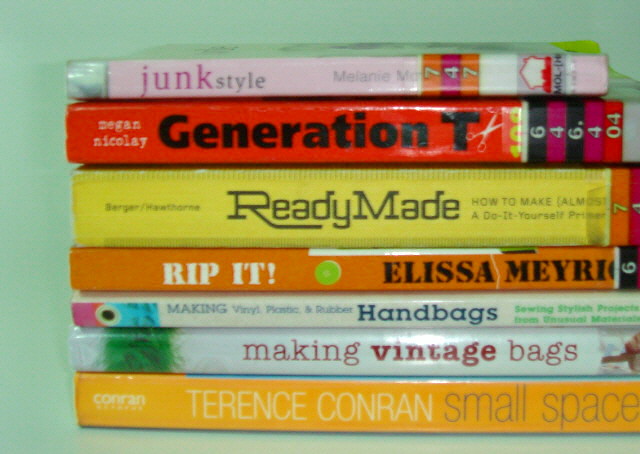This image depicts a neatly stacked collection of seven books, each with its title clearly visible on their spines, set against a green background. Starting from the bottom, the titles are: "Small Space" by Terrence Conran, distinguished by a yellow spine; "Making Vintage Bags" on a white spine with red lettering; "Making Vinyl, Plastic, and Rubber Handbags," also on a white spine but with blue text; "Rip It" by Elisa Mebryk on an orange spine; "Ready Made: How to Almost Do It Yourself" on a thick yellow spine; "Generation T" on a red spine; and finally, "Junk Style" on a pink spine at the very top. The books are aligned in such a way that only their bindings are visible in the photograph, with the right edges of the bindings cropped off slightly. The green background provides a striking contrast to the vivid colors and diverse titles of the book spines.